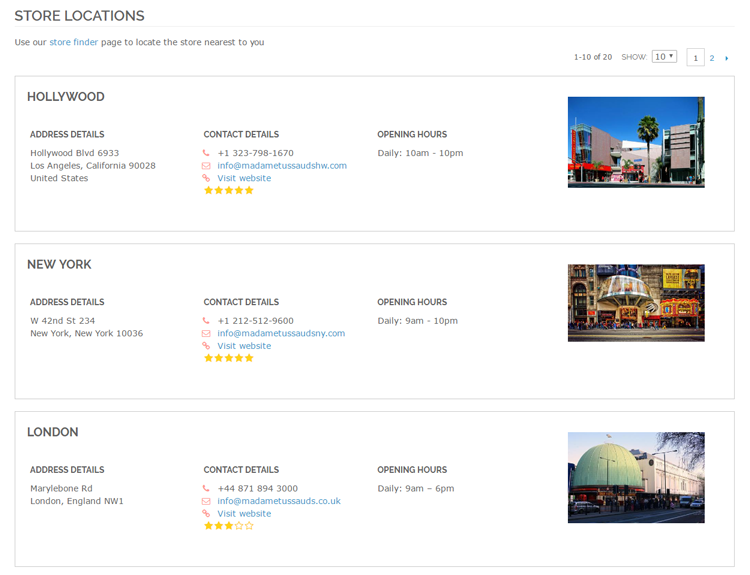The screenshot is taken from a website, featuring a white background with gray font. At the upper left corner, it reads "Store Locations," followed by a smaller font note: "Use our store finder page to locate the store nearest to you." The page lists three store locations with detailed information for each.

1. **Hollywood:**
   - **Location:** Hollywood
   - **Address Details:** Specific address (details provided)
   - **Contact Details:** Phone number, email address, and website
   - **Ratings:** Five gold stars indicating very high customer ratings
   - **Opening Hours:** Daily from 10 a.m. to 10 p.m.
   - **Photo:** Image depicting two storefront buildings on opposite sides of the street, with a large palm tree and blue skies in the background.

2. **New York:**
   - **Location:** New York
   - **Photo:** The image includes some orange elements, likely part of a storefront.

3. **London:**
   - **Location:** London
   - **Photo:** Displays a distinctive dome-like shape close to the ground with a light green color.

Each store listing includes address and contact details, high customer ratings indicated by gold stars, and their respective opening hours. The right side of the webpage showcases a photo corresponding to each store location, providing a visual context of the area.